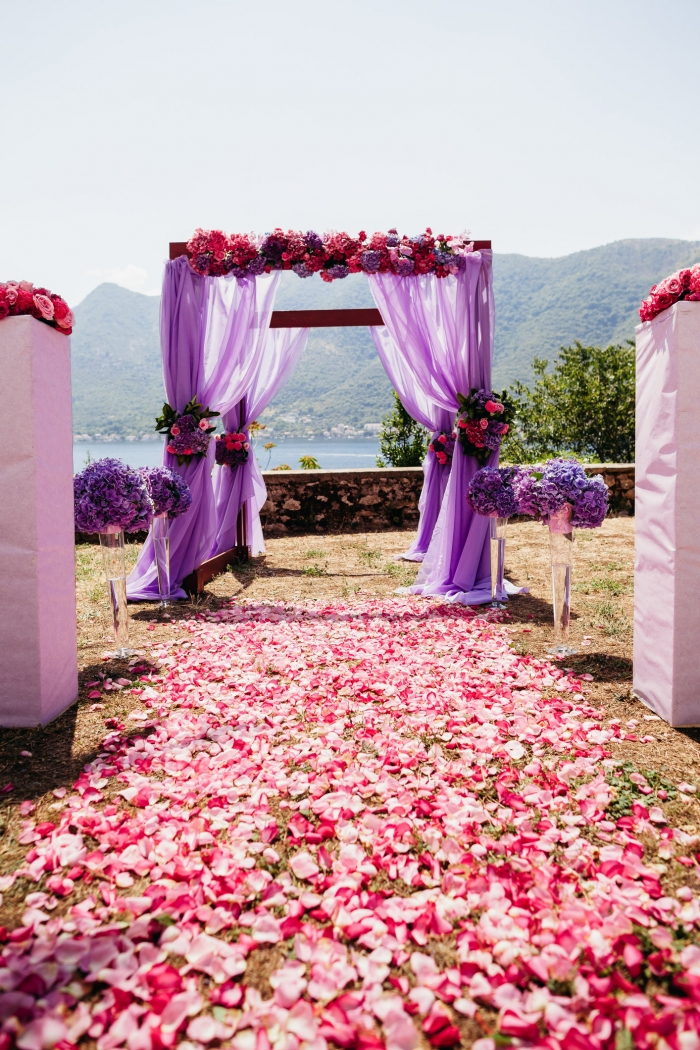The photograph showcases a picturesque outdoor wedding setup. The ground is adorned with a pathway of white and pink rose petals leading to a charming wooden canopy structure. This canopy, resembling a gateway, features a square frame with four legs draped in lavender-colored sheer curtains tied back with bundles of pink flowers and green leaves. The crossbeam at the top of the canopy is also decorated with bouquets of flowers. The wedding aisle, bordered by additional decorative items and flanked by columns that likely mark the seating areas, is a grassy expanse with intermittent brown patches. In the background, a small stone retaining wall frames the scene, beyond which lies a serene body of water and distant rolling hills under a clear sky. The entire scene exudes a romantic and idyllic atmosphere, perfectly set for a wedding ceremony.